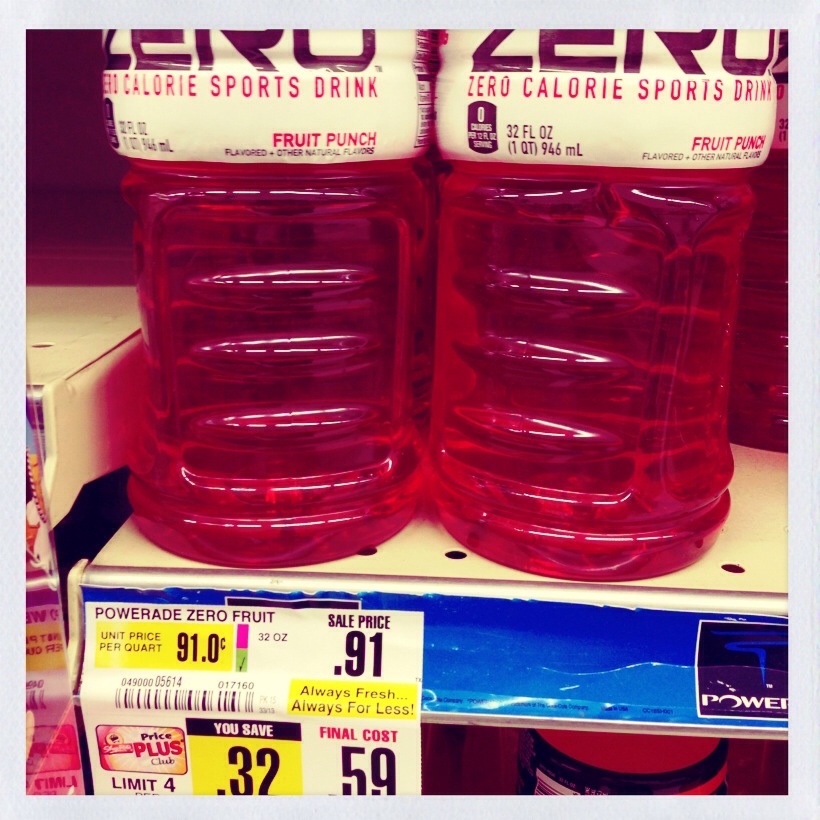The image is a square photograph featuring a close-up of a store shelving unit, bordered by a very light gray, thin edge. Dominating the frame is a banner affixed to the side of the shelf displaying a price tag for "Powerade Zero Fruit," on sale for $0.91. Above this banner, the shelf holds two bottles of Powerade Zero, positioned side-by-side horizontally. The photograph captures only the bottom halves of these bottles. The labels on the bottles show the word "Zero" in purple on a distinct white background. Below in bold red text, the label reads "Zero Calorie Sports Drink," followed by the flavor designation, "Fruit Punch." The lower half of the bottle's content is encased in clear plastic, revealing the vibrant red color of the Fruit Punch beverage. This detail-rich image highlights the promotional pricing and the design elements of the Powerade Zero product.